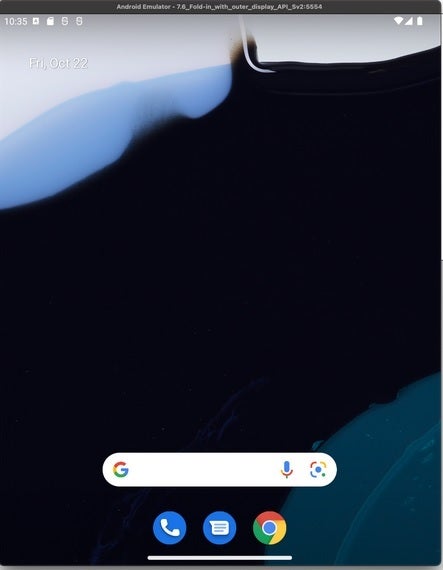This image is a detailed screenshot of an Android emulator's homepage. At the top of the screen, a small font indicates that the device in question is an Android emulator, not a physical phone. It's clearly not an iPhone, suggesting it might be a Google phone or another type of Android device. The time displayed in the top left corner reads 10:35, though it is unclear if this is a.m. or p.m. 

On the right side of the status bar, several icons display the device's status: full cell signal strength, strong Wi-Fi connectivity, and a fully charged battery at 100%. The date is prominently shown as Friday, October 22nd. 

The background image is a prominent abstract artwork featuring a large, undefined black swatch in the center, surrounded by light blue and gray hues, making it indiscernible what the picture represents.

Centrally positioned at the bottom, there is a Google search bar for quick web queries. Below the search bar, several key icons are visible: a telephone icon for making calls, a text message icon for sending messages, and the familiar Google Chrome icon to access the web browser.